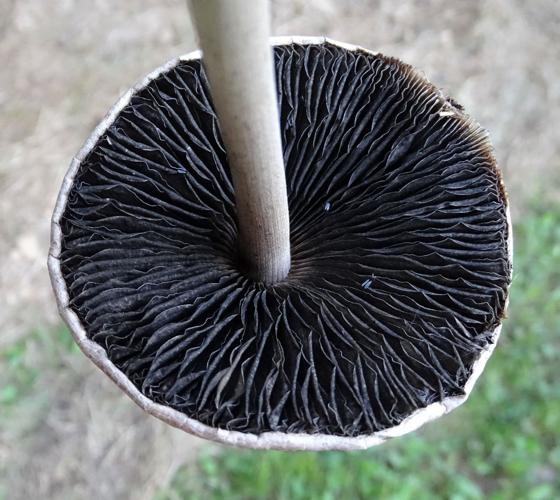This photograph captures an intimate view of the underside of a mushroom. Dominating the composition, the white stem descends gracefully from the top center, terminating in the middle of the frame. Encircling the stem, the underside of the mushroom cap is prominently displayed, characterized by its intricate, black, crinkly structure reminiscent of delicate, crumpled paper. Slight hints of the mushroom's white dome crown the edges of this organic tapestry. In the background, a blur hints at elements of a natural setting; the bottom right quadrant reveals some grass, while the remaining areas suggest rocky terrain. The image artfully focuses on the distinct textures and subtle contrasts of the mushroom's underbelly.